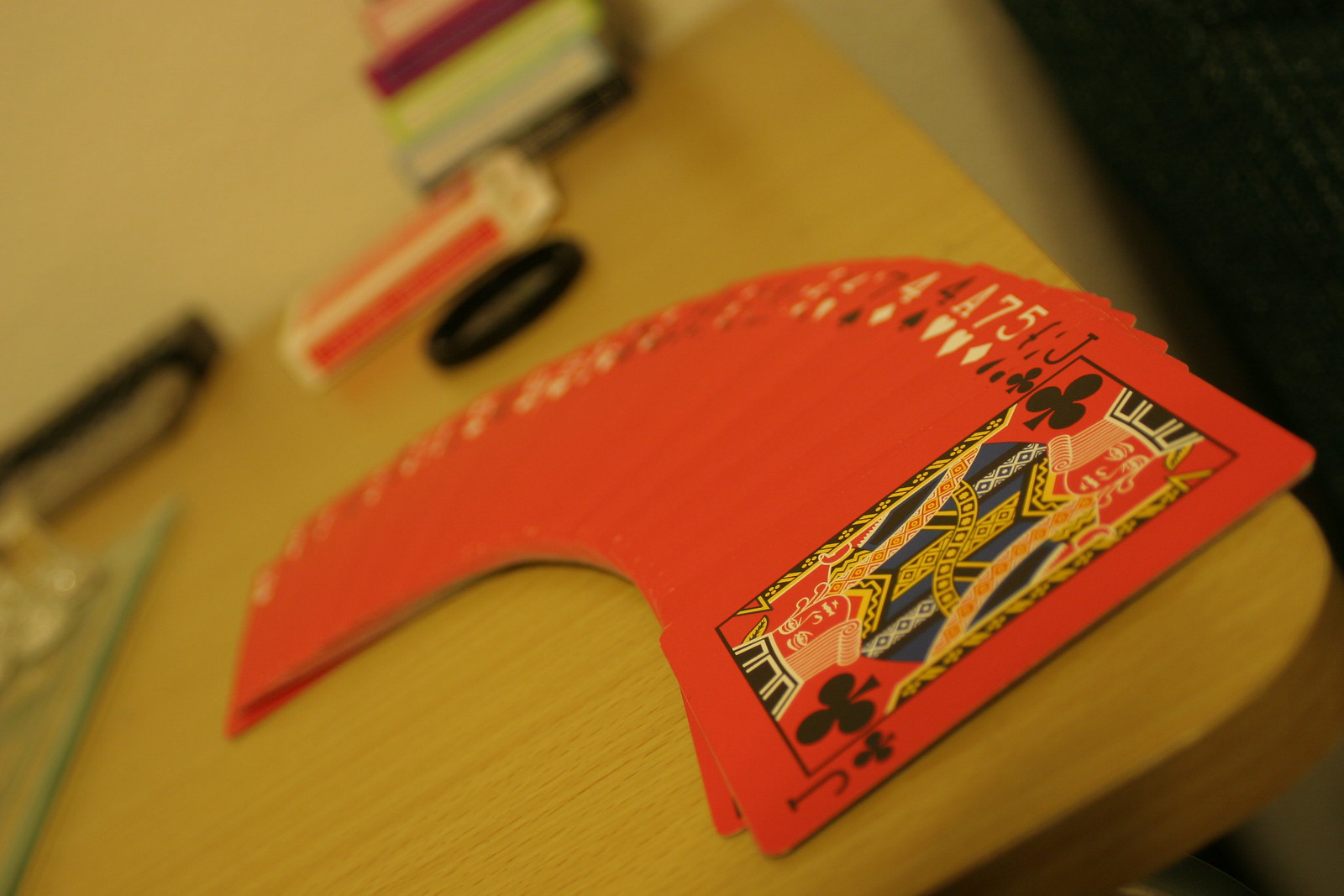In this partially blurry image, the main focus is on the corner of a table situated in the bottom right corner of the frame. Sprawled across this corner are neatly spread playing cards, reminiscent of a magician's display before a card trick. These cards are face up and exhibit a red design on their fronts. Dominating the spread is a Jack of Clubs, conspicuously black, followed by a Five of Diamonds, with diamonds and numbers uniquely in white instead of the traditional red. Positioned slightly beyond the cards is a presumed coaster, adding a subtle detail to the scene. To the right, a slightly visible cushion, possibly part of a couch, adds context to the setting. Also present, but equally blurry, is the box from which the cards originated, flanked by a stack of three or four indistinct books.